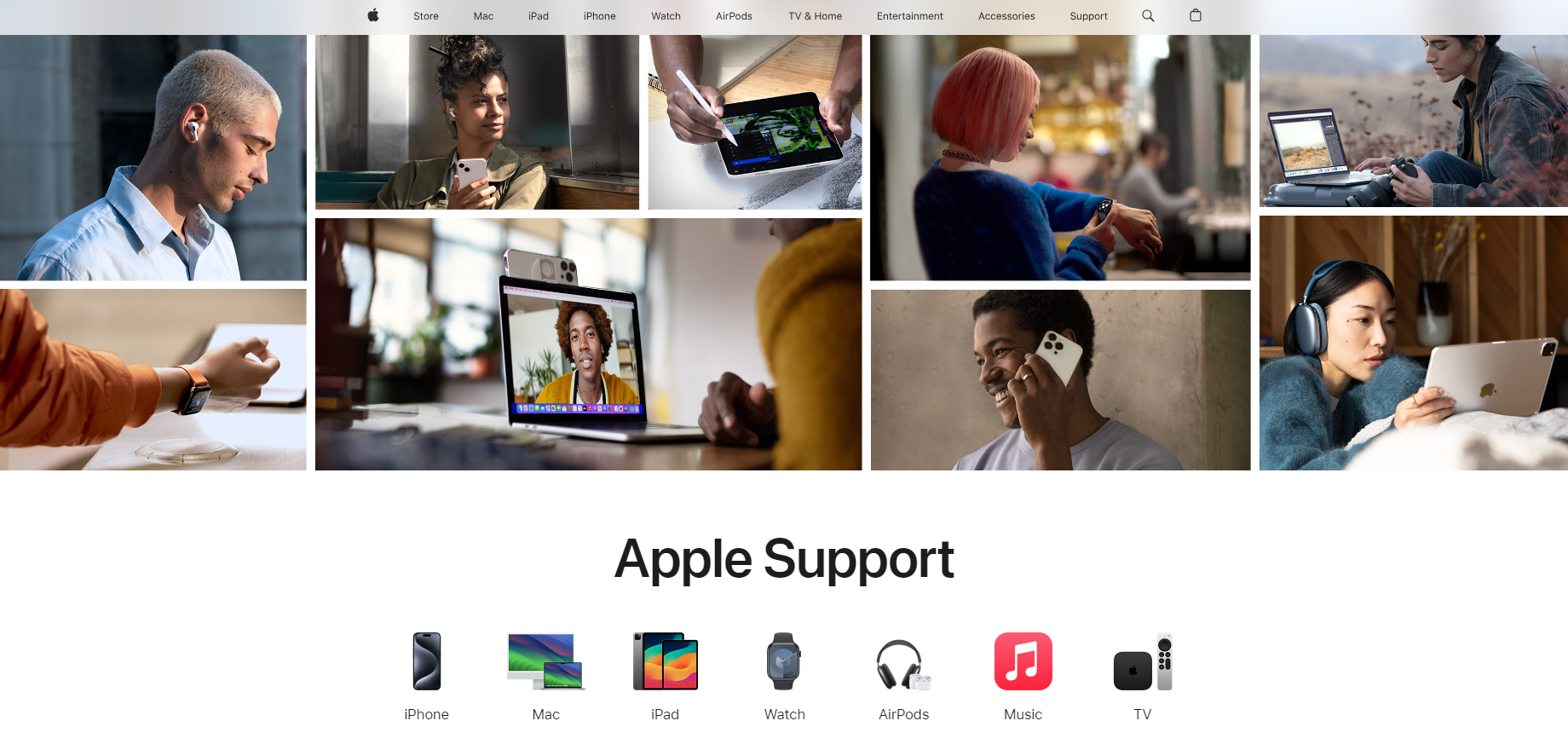This image captures a screenshot from a computer screen displaying the Apple website. The familiar Apple logo is prominently positioned in the top left corner. The header features a gray background and includes clickable text options arranged horizontally: Store, Mac, iPad, iPhone, Watch, AirPods, TV & Home, Entertainment, Accessories, and Support. Additionally, there is a magnifying glass icon for search functionality and a shopping bag icon for the cart.

The main section of the screen is divided into a grid of images. At the top, there are five images, and below them, four images occupy larger spaces, creating an asymmetrical arrangement. These images depict various Apple products and users, including individuals wearing AirPods and headphones, engaging with the technology. Beneath the images, text reads "Apple Support" beside icons representing iPhones, iPads, and other miscellaneous Apple products. The website's design effectively showcases Apple's diverse product lineup and emphasizes user engagement with its technology.